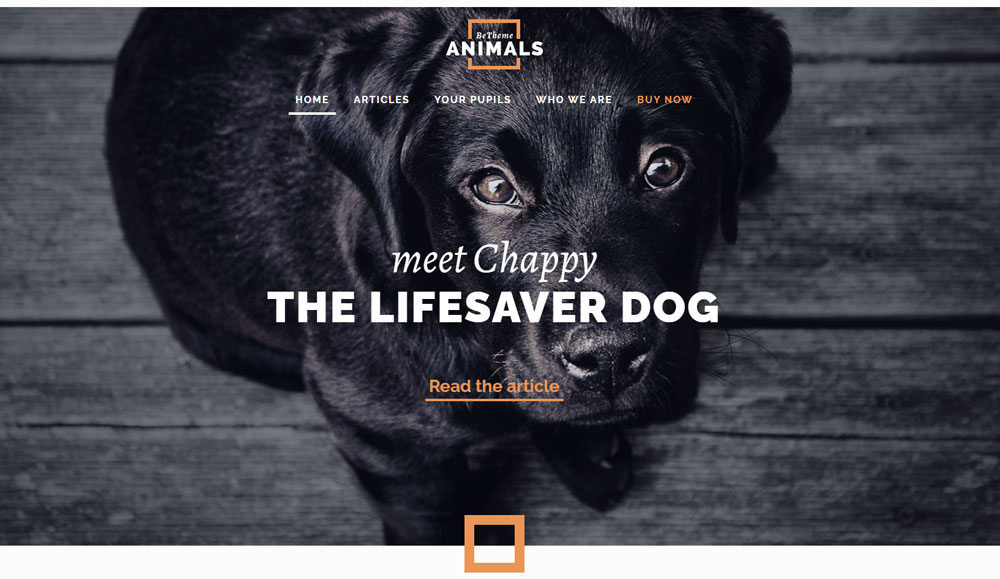The image titled "Bee-Themed Animals" features a captivating scene centered around a large, endearing dog named Chappy. The background consists of a mixture of gray and wooden flooring, providing a cozy atmosphere. Chappy, the lifesaver dog, is portrayed with expressive, soulful brown eyes and a slightly wet black nose. His fur is a blend of brown and black tones, enhancing his warm and gentle appearance.

The text "Bee-Themed Animals" is written in white within the image, though "bee-themed" is smaller and encased in a white rectangular outline. The rectangle intriguingly intersects the word "animals," starting at the letter 'N,' extending downward and to the right, curving back up near the 'L,' then moving left and back down to the 'N.'

A menu path spans across the top of the image, listing options such as "Home," "Articles," "Your Pupils," "Who We Are," and a prominently highlighted "Buy Now" in orange, signifying it is currently selected. The main headline reads, "Meet Chappy, the Lifesaver Dog," encouraging viewers to "Read the Article," with the latter phrase being an orange clickable link.

Additionally, near Chappy's left paw, there is a small orange square positioned slightly towards the center of the image, adding a subtle focal point near the bottom left of the dog's paw. This thoughtful arrangement of elements draws attention to Chappy's story while maintaining a visually engaging composition.